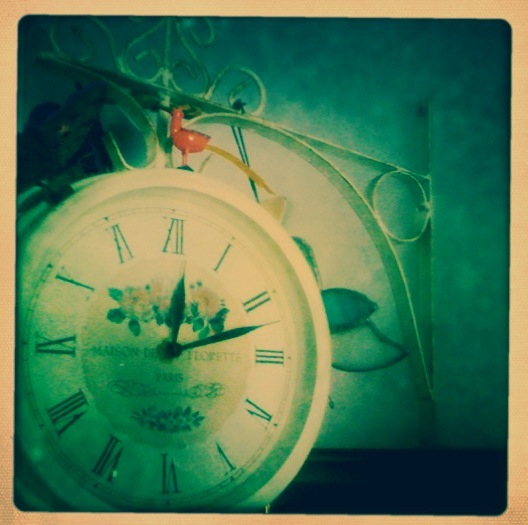This image appears to be a screenshot from a video game, depicting a scene reminiscent of a vintage Polaroid photograph but with a narrower, tan border. In the bottom left-hand corner, there is an antique clock adorned with Roman numerals and decorated with an array of colorful flowers at its center. The clock hands indicate a time slightly past 12:10, around 12:13. 

Behind the clock, occupying the upper left portion, is a blackish figure that seems to be a crow, though its details are difficult to discern. Atop this figure, there's a small, red trinket that vaguely resembles a miniature toilet with legs, adding a quirky element to the composition.

The background features a white wrought iron structure, possibly part of a bed frame or another piece of ornate furniture, with swirling and looping designs. The image exhibits a gradient of color, with the central portion taking on a teal-ish blue hue, which gradually darkens to a deeper blue towards the edges. The overall appearance of the image is intentionally blurred and aged, contributing to its vintage aesthetic.